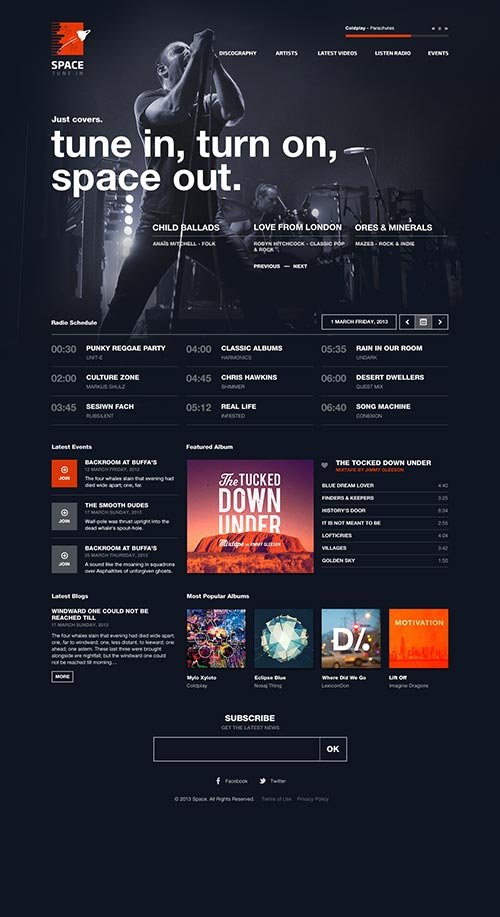### Space Radio Station Homepage

**Logo and Navigation:**  
At the top left of the homepage, the Space logo is prominently displayed next to the text "Space," emphasizing the brand name. On the top right, there are two key navigation links: "Catalog" and "Partnerships."

**Main Visual and Slogan:**  
The homepage features a striking black and white image of a musician performing passionately on stage. Overlaid on this image is the evocative slogan: "Tune In, Turn On, Space Out."

**Music Categories:**  
Below the main slogan, three distinctive music categories are highlighted: 
- Child Ballads
- Love from London
- Ores and Minerals

**Radio Schedule:**  
A detailed radio schedule is displayed, starting from 2:00 PM:
- 2:00 PM: Punny Reggae Party
- 2:40 PM: Culture Zone
- 3:45 PM: Szechuan's Fac
- 4:00 PM: Classic Albums
- 5:12 PM: Real Life
- 6:30 PM: Rain in Our Room
- 7:00 PM: Desert Dwellers
- 8:40 PM: The Song Machine

**Events and Albums:**  
The "Latest Events" section lists upcoming events with dates, venues, and brief descriptions, such as performances by "Backroom at Buffa's" and "The Smooth Dudes."

A "Featured Album" section showcases the album "Tucked Down Under," including artwork and a tracklist with songs like:
- The Blue Dawn Lover
- Prince and Warrior
- History's Book
- It's Not Meant to Be
- Villages
- Golden Sky

**Blog Features:**  
The blog section features expert articles with intriguing titles, such as "Window One Could Not Be Reached Till."

**Popular Albums:**  
A selection of popular albums is displayed with thumbnail covers, including:
- Emoji
- Xylus
- Eclipse
- Ethano
- When Did We Go
- Lil' Or

**Subscription and Social Media:**  
A subscription box invites users to stay updated with the latest news. Social media icons for Facebook and Twitter are easily accessible.

**Footer Links:**  
The footer contains essential links to the terms of service, privacy policy, and other relevant legal information.

**Overall Design:**  
The website has a sleek, modern design, with an emphasis on music content. It provides easy access to radio schedules, events, albums, and blog posts, ensuring a user-friendly experience for music enthusiasts.